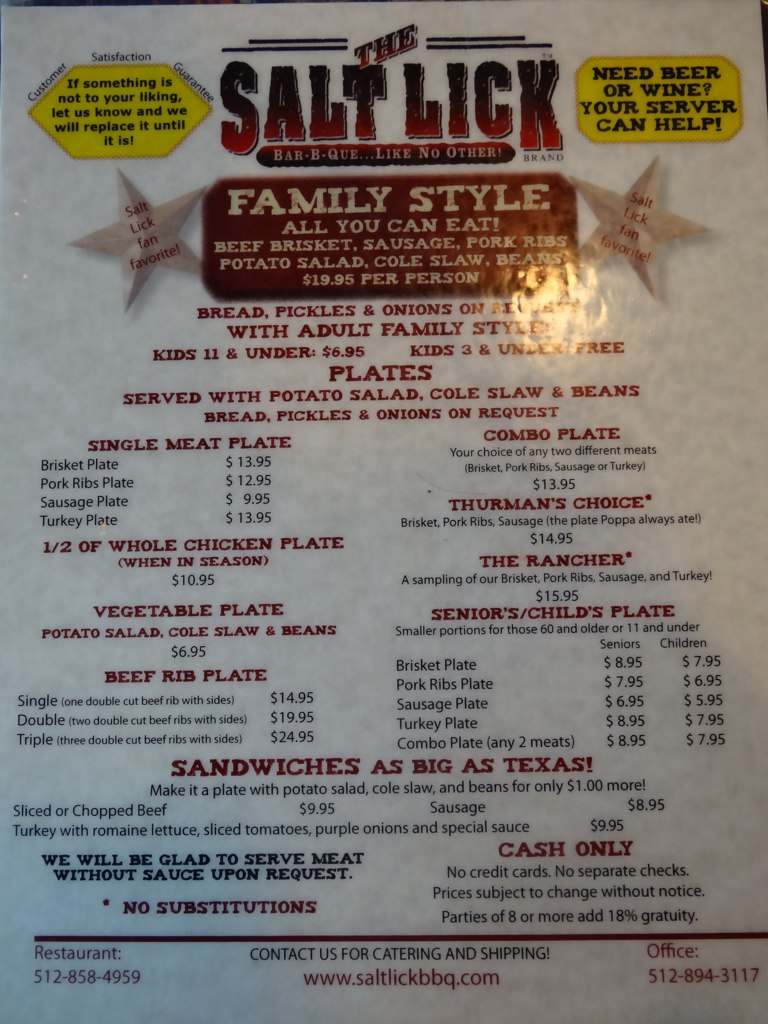This photograph captures the surface of a menu from The Salt Lick BBQ, encased in a clear plastic cover within a holder. The top-right area of the image is marked by the circular reflection of a camera flash or overhead light fixture. The menu prominently displays the restaurant’s name, "Salt Lick," followed by the tagline "BBQ like no other, family style." 

The menu details various plate options, all of which include potato salad, coleslaw, beans, and optionally, bread, pickles, and onions. The offerings range from single meat plates to combinations, half and whole chicken plates, specialty options like Thurman's Choice and The Rancher, a vegetable plate, senior and child’s plates, and a beef rib plate. The menu also mentions the sandwiches, described as "big as Texas."

Pricing is detailed, with most plates in the $13-$14 range, The Rancher priced at $15.95, and the vegetable plate at $6.95. An additional note in the upper-right corner mentions that servers can assist with beer and wine requests. The contact information provided includes two phone numbers, 512-858-4959 and office 512-894-3117, along with the website address, www.saltlickbbq.com. The overall presentation underscores the advertisement and pricing details for the offerings of The Salt Lick BBQ.